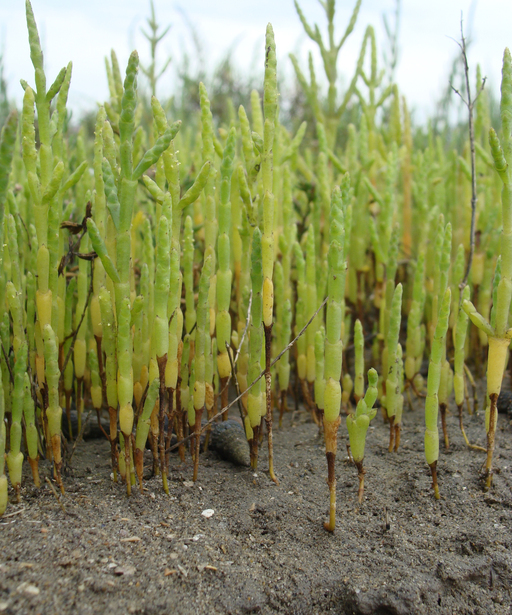This image is a detailed close-up of tall, straight, green plants that appear to be some form of segmented vegetation, possibly succulent-like or resembling cacti. Each plant stands several feet high with a predominantly straight, vertical growth, occasionally branching off at angles but still pointing upwards. The plants exhibit a range of green hues, from light to dark, with some sections having a yellowish tint.

The plants grow closely together in a moist, dark, sandy soil, which appears grayish-brown to black and contains small rocks and debris. The soil's wetness is evident from its darker coloration. In the background, a vague brown mass is partially visible, suggesting the image includes an outdoor setting on a bright, sunny day. The focal point remains on these distinctive green plants with their segmented, slightly rounded sections contrasting sharply against the darker, textured soil.